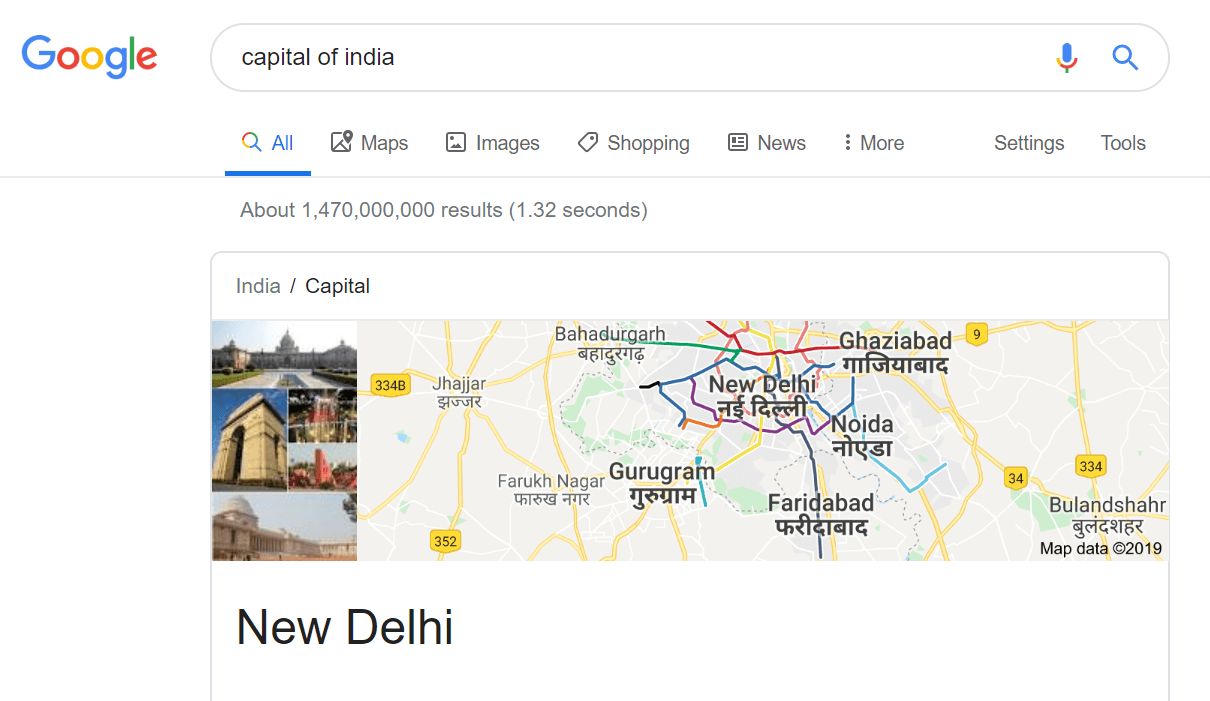A Google search for "capital of India" displays results highlighting New Delhi. The main search page offers options to explore Maps, Images, Shopping, News, and more settings and tools. The search yields approximately 1 billion 470 million results in just 1.32 seconds. At the top, "India / Capital" is displayed, with "New Delhi" prominently highlighted in large, bold black letters. The page showcases various photographs of New Delhi, depicting different parts of the capital city. 

In addition, a detailed map is presented at the center, clearly marking New Delhi and its surrounding areas. Key streets are highlighted in yellow, with street and route numbers prominently displayed within yellow circles for easy navigation. The map provides an overview of neighboring towns as well. The information is presented bilingually, featuring both English and the native language, facilitating accessibility for a diverse audience.